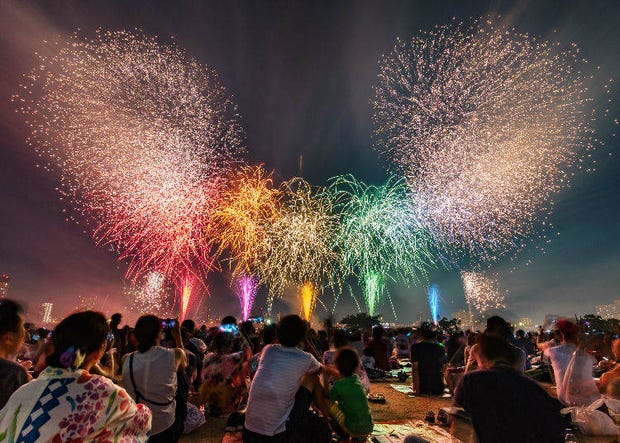The image captures a dazzling firework display lighting up the night sky with vibrant colors. At the center of the photograph, five differently colored fireworks explode magnificently, with hues of red, purple, yellow, green, and blue streaking across the sky. Glittery white fireworks bookend the colorful display on either side, creating prominent large sparkling bursts. Below the fireworks, a crowd of people sits on a tannish-colored surface, their backs turned towards the camera, dressed in a variety of colored clothes including greens, reds, whites, and blacks. They appear to be seated on some kind of fabric material laid on the ground. The sky above is a dark gray, indicative of the evening setting, with distant, blurry buildings with lights faintly visible around the edges. The main focus of the image is clearly the vivid fireworks, with their streams of color ascending into the sky and exploding into beautiful, radiant patterns, overshadowing the less distinct surroundings.